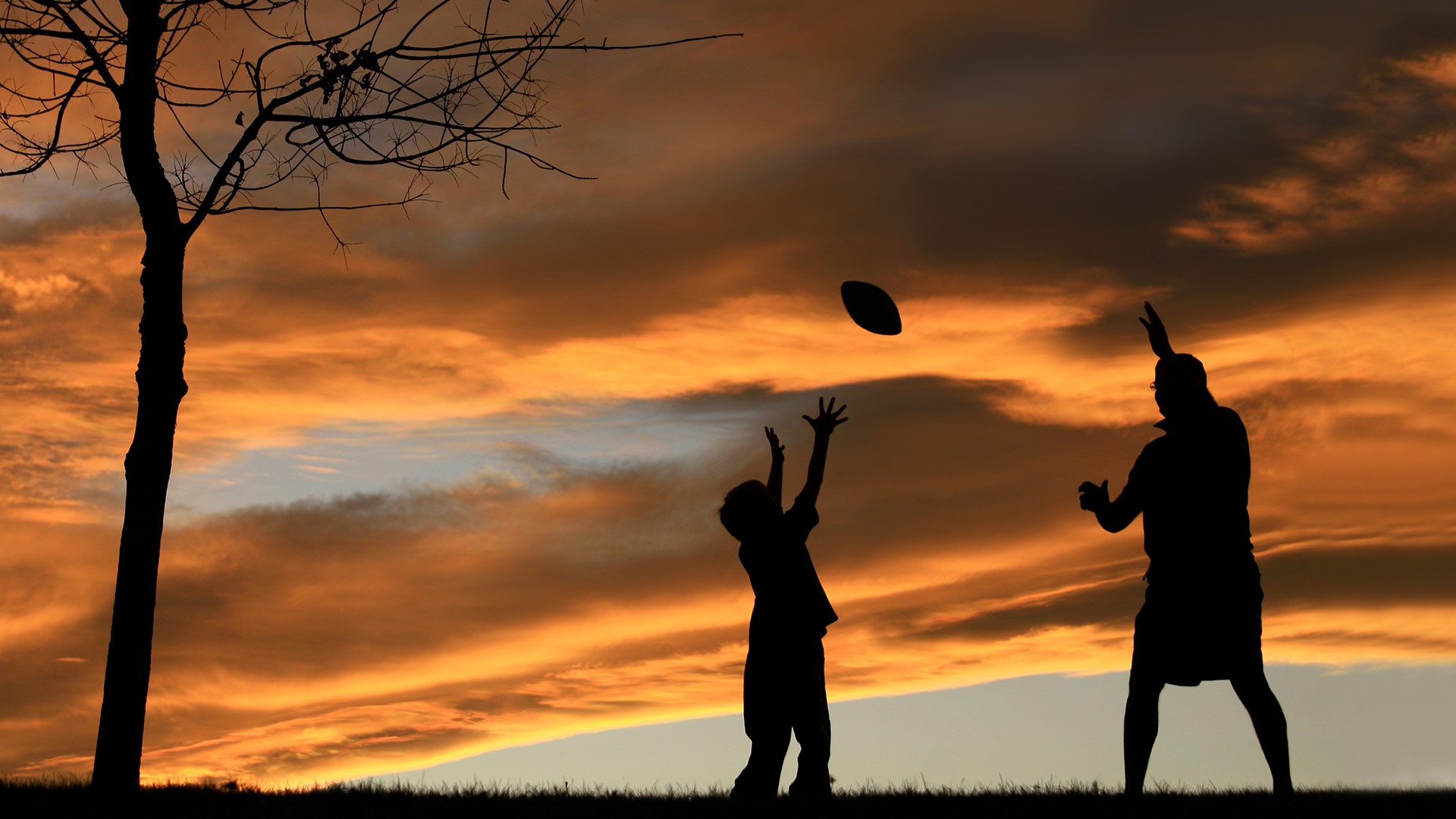This captivating photograph, likely taken at sunset, showcases the silhouetted forms of a man and a young boy engaging in a heartfelt game of football outdoors. The rectangular image, approximately six inches wide by three inches high, captures a serene evening scene with the sun already below the horizon. 

In the lower eighth of the image, the crest of a hill appears in stark black shadow, dotted with faint, shadowed grass. To the left, the barren trunk of a tree stretches from the bottom to the top of the frame, with a few remaining dead leaves clinging to its upper branches.

On the right side of the image, the man, legs shoulder-width apart, is captured in mid-throw, his arms dynamically positioned: one extended forward and the other aloft. The young boy stands to his left, arms raised in anticipation of catching the arcing football above him. 

Above this lively scene, the sky is a stunning gradient of gray, transitioning to a vibrant display of glowing reds, oranges, and creamy yellows that tint the bottom of large, dark gray clouds which dominate the upper part of the image. The entire scene is bathed in the soft, diffused light of the setting sun, accentuating the silhouettes and lending a dreamy quality to the moment frozen in time.